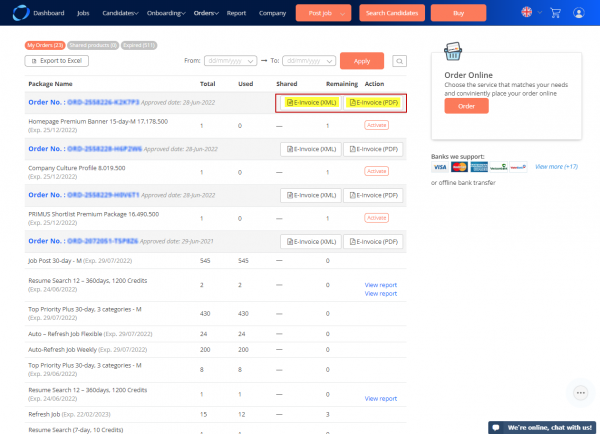A detailed view of the computer screen displays a segmented interface with distinct sections and features. In the top left corner, the screen prominently shows the word "Dashboard" against a dark blue background. Here's a breakdown of the interface:

1. **Top Navigation Bar**:
   - **Left Side**: Dark blue background with "Dashboard" clearly visible.
   - **Right Side**: Regular blue background with a list of options in white text on a salmon pink background. These include "Find Job," "Search Candidates," and "Buy." Additionally, an English flag icon, a card icon, and a profile icon are neatly aligned on the far right.

2. **Main Categories**:
   - Below the top navigation, the interface divides into six main categories, each label in white text: "Jobs," "Candidates," "Onboarding," "Orders," "Report," and "Company."

3. **Data Section**:
   - The data table below these categories includes columns titled: "Package Name," "Total," "Used," "Shared," "Remaining," and "Action." Each of these columns is populated with corresponding data. Four entries in the "Order Numbers" column are displayed in blue text, while other cells contain black text or dashed lines indicating missing information.

4. **Service Information**:
   - On the right-hand side, the section titled "Order Online" encourages users to "Choose a service that matches your needs and conveniently place your order online," accompanied by an orange "Order" button.

5. **Additional Services**:
   - Below, a section labeled "Banks We Support" lists some popular banks, highlighting the platform's versatility and support for various financial institutions.

6. **Customer Support**:
   - In the bottom right corner, a dark blue logo provides the prompt "We're Online, Chat With Us," offering real-time assistance to users.

The detailed layout and strategic color usage ensure that the interface is user-friendly and the actionable items are readily accessible.